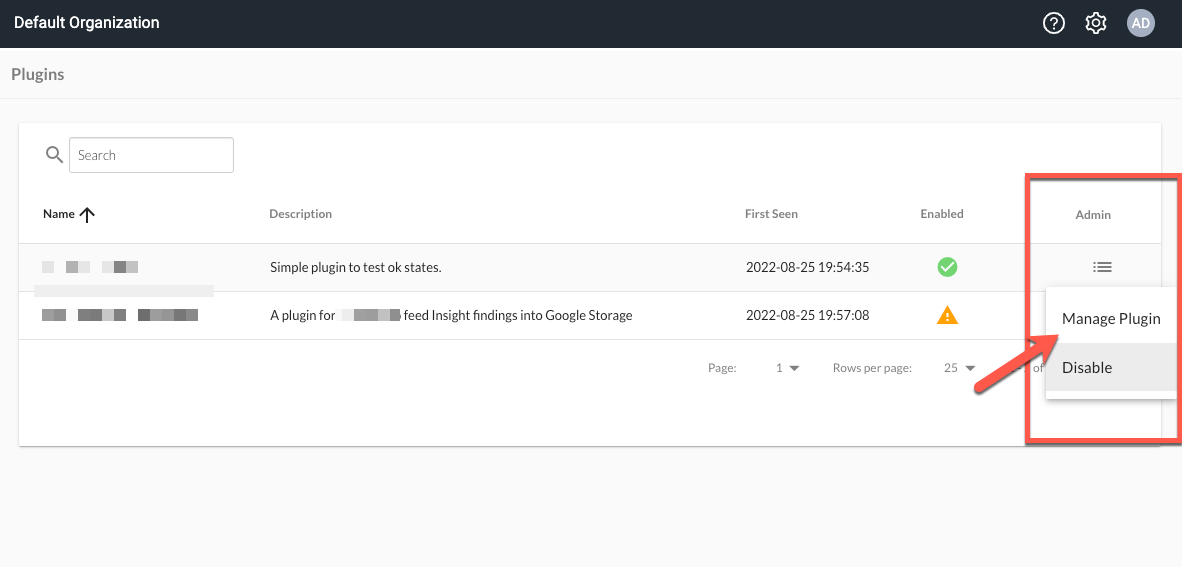In this image, the topmost section features a black bar with white text on the left that reads "Default Organization." On the right side of this bar, there are three icons: a question mark for help, a settings gear icon, and a user icon labeled "AD." Beneath this bar, on the left, there's the word "Plugins" in gray text, followed by a search box containing a small magnifying glass icon but no text. Below the search box, there are various lines of information organized into columns with the following headers: "Name," "Description," "First Seen," "Enabled," and "Admin."

In the "Name" column, the text is digitally obscured, making it unreadable. In the "Description" column, there are two entries: "Simple plug-in to test" and "plug-in for [digitally altered text] feed insight findings and to search Google storage." 

Finally, in the "Admin" column to the far right, there is a red square with an arrow pointing toward a "Manage Plugin" option.